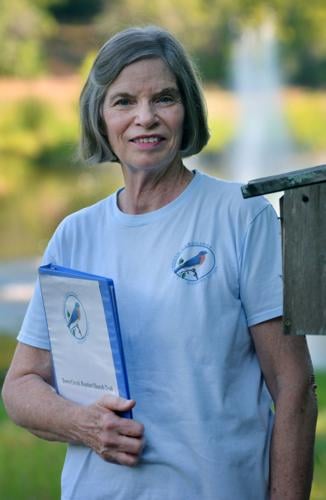This photograph features an elderly woman, possibly in her 70s, with a joyful smile displaying her teeth. Her short, grayish-brown hair is styled in a bob, slightly pulled back on one side. She sports a light blue t-shirt adorned with a bird emblem on the chest, which matches the same bird emblem on the cover of the blue binder she is holding. The scene captures her leaning against a wooden birdhouse, possibly at a bird sanctuary or nature preserve. In the blurred background, a water fountain sprays amidst green trees and fields, further suggesting the natural setting. Her pink lipstick adds a touch of color to her cheerful demeanor, and while no live birds are visible, the bird emblems on her attire hint at a connection to avian care or bird watching.